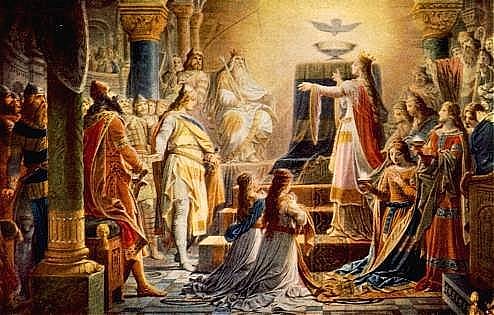The scene is a vibrant, illustrative painting showcasing a Middle Ages throne room filled with a diverse assembly of people. The rectangular image, about three to four inches wide and two inches high, depicts an old and ornate indoor setting. Central to the scene, a series of stone steps ascend to a simple yet elevated throne. Seated on this throne is an older man with a long white beard and hair, adorned with a crown and holding a scepter that rests on his right shoulder. Adjacent to him, atop the throne, is a statue of an eagle, adding to the regal ambiance.

Two young women in white gowns, one with a blue sash and the other with a red sash, are kneeling on the stone floor at the foot of the steps, their long hair cascading down to their waists. To the left of the image, two painted columns—one green and one blue with a gold top—frame a group of bearded men dressed in medieval cloaks and armor. Beside them, there are numerous individuals donning long flowing robes, hats, and capes typical of Middle Ages attire.

Towards the right side of the painting, primarily women gather, their attention focused on the central throne and the kneeling figures. Apart from the throne, an altar features prominently, topped with a bowl and a dove above it, emanating a bright light possibly symbolizing the Holy Grail. This detailed and evocative scene captures the richness and ceremonial splendor of a medieval court.